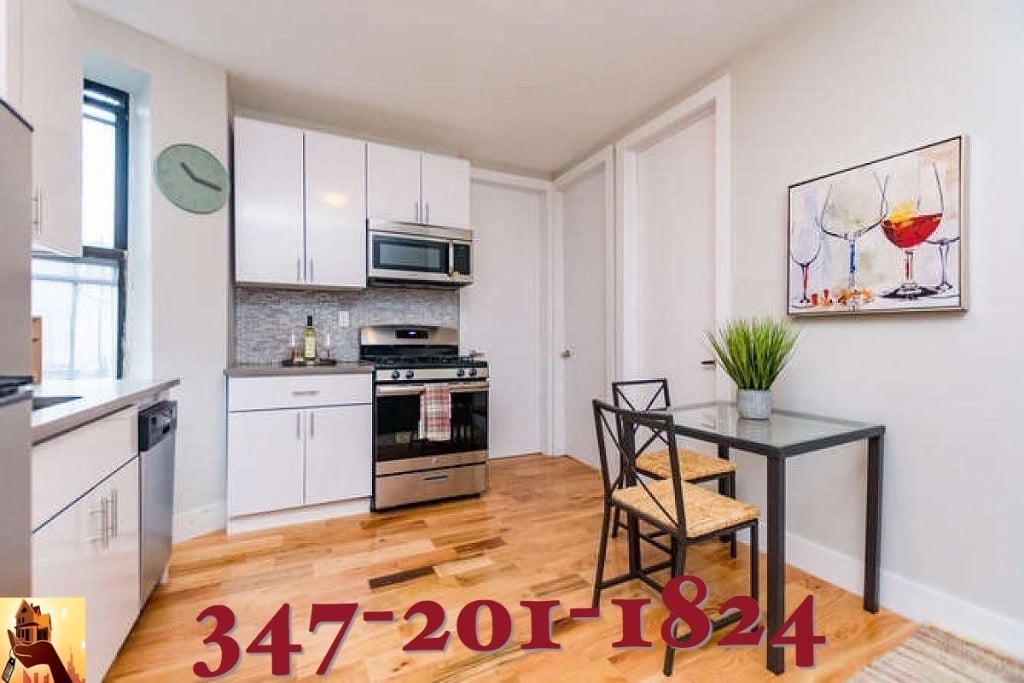This image is a meticulously styled advertisement showcasing the kitchen and dining area of a home or apartment available for rent. Central to the scene is a pristine kitchen outfitted with sleek white cabinets featuring minimalist white handles. Key appliances, including an oven, microwave, and sink, are positioned within the cabinetry, accentuating the clean and modern design.

The dining area, located on the right side of the image, boasts a contemporary glass table with black legs, accompanied by two chic chairs. A large potted plant serves as an attractive centerpiece, adding a touch of nature to the setting. Above the dining table hangs an elegant framed picture of various wine glasses, contributing to a sophisticated ambiance.

The room is adorned with light brown wooden flooring that complements the white walls and ceiling, enhancing the bright and airy feel of the space. A large blue clock in the top left corner adds a pop of color and functionality. Natural light streams in through the windows, further highlighting the immaculate condition of the area.

To facilitate inquiries and rental prospects, a prominent red phone number, 347-201-1824, is displayed at the bottom center of the image, directed towards potential tenants seeking more information.

Overall, the image exudes a welcoming and stylish atmosphere, effectively appealing to prospective renters.